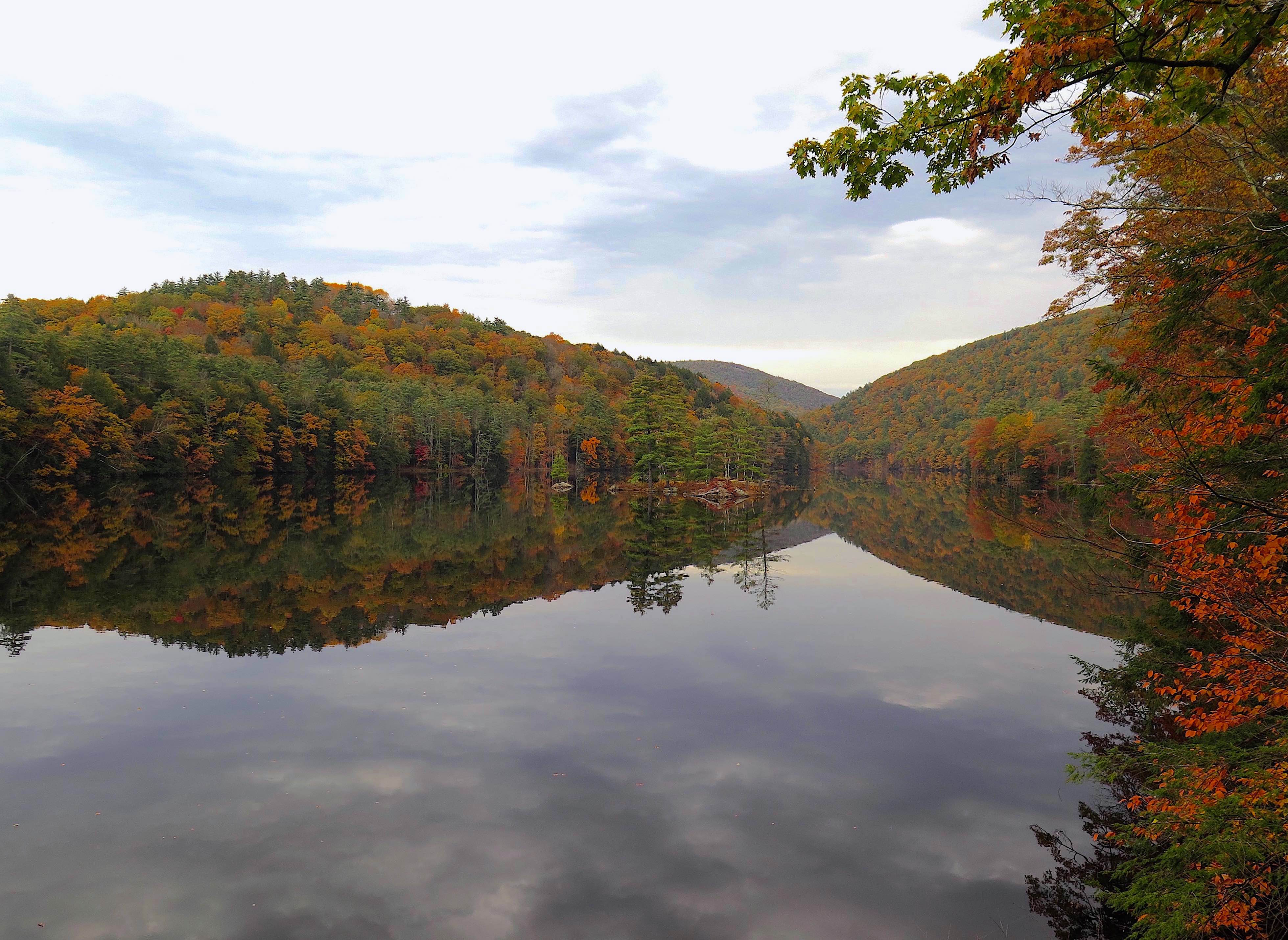This stunning landscape photograph, likely taken in early autumn in New England or another region with distinct seasons, captures a serene mountain lake. The lake, appearing almost as still as glass, beautifully reflects a sky adorned with wispy, white clouds. Stretching over a large area, the lake's tranquil waters perfectly mirror the surrounding scenery. In the distance, gently rolling hills and mountains envelop the lake, their slopes covered in forests showcasing a symphony of fall colors, including vibrant reds, oranges, yellows, and greens. 

In the foreground on the right stands a striking tree adorned with orange and red leaves, its branches extending gracefully over the lake. This overhanging branch, along with the distant hills and foliage, is vividly reflected in the calm water, creating a harmonious, peaceful scene. The composition highlights the crispness of the season, emphasizing the natural beauty and stillness of the lake and its picturesque surroundings.